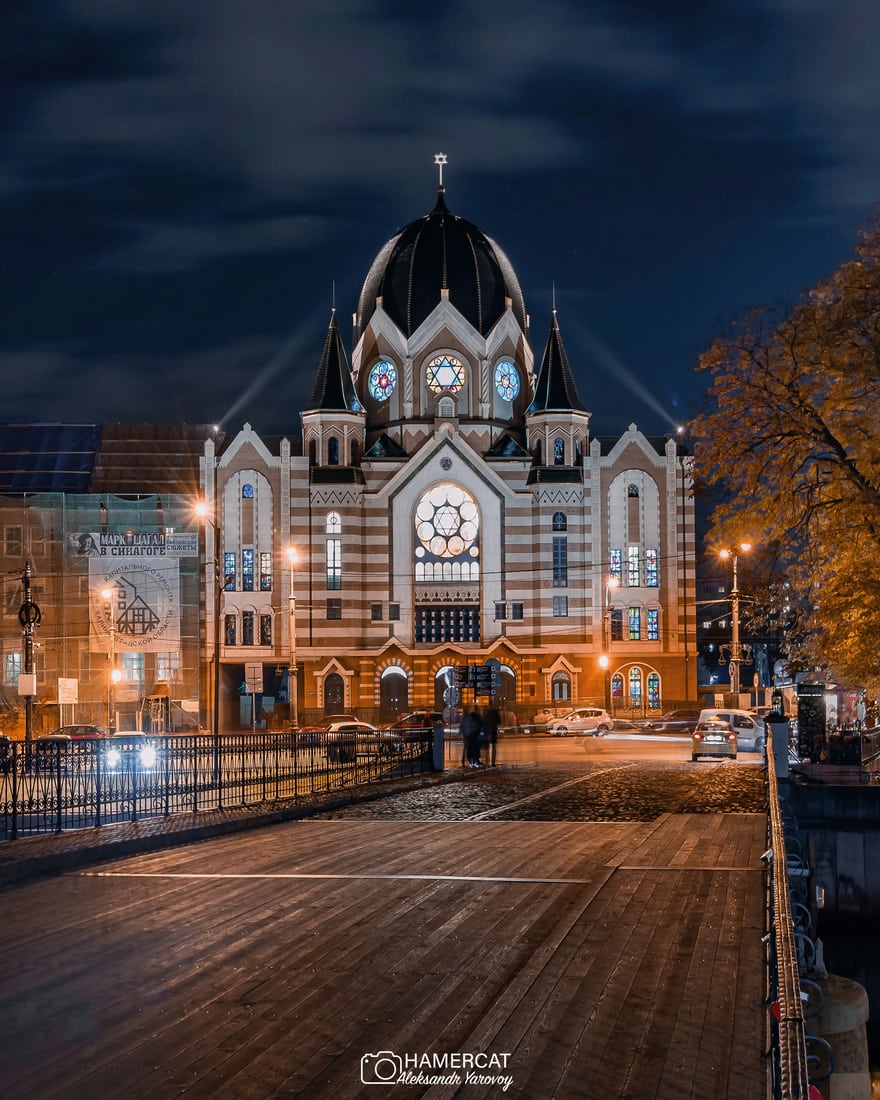The image, taken at night, showcases a grand, Russian-style building with a prominent dome roof that curves up and is black in color. At the top of the dome, there is a silver ornament. The dark blue night sky features a few clouds, adding to the atmospheric scene. Spotlights illuminate the dome, which is complemented by two spires on either side. Below the dome, three stained glass windows are visible, featuring a Jewish star on one of them. The building's facade displays a mixture of light and medium brown bricks with horizontal white stripes, giving it a unique architectural appeal that hints at a Gothic influence. The large stained glass window above the entrance is especially eye-catching. In front of the building, the road, which appears to be part wood and part cobblestone, has several cars parked along it. There is also an adjacent building to the left. The image bears a watermark indicating "hammer cat" with an icon of a camera. Orange lights shine from the sides of the building, enhancing its majestic appearance.